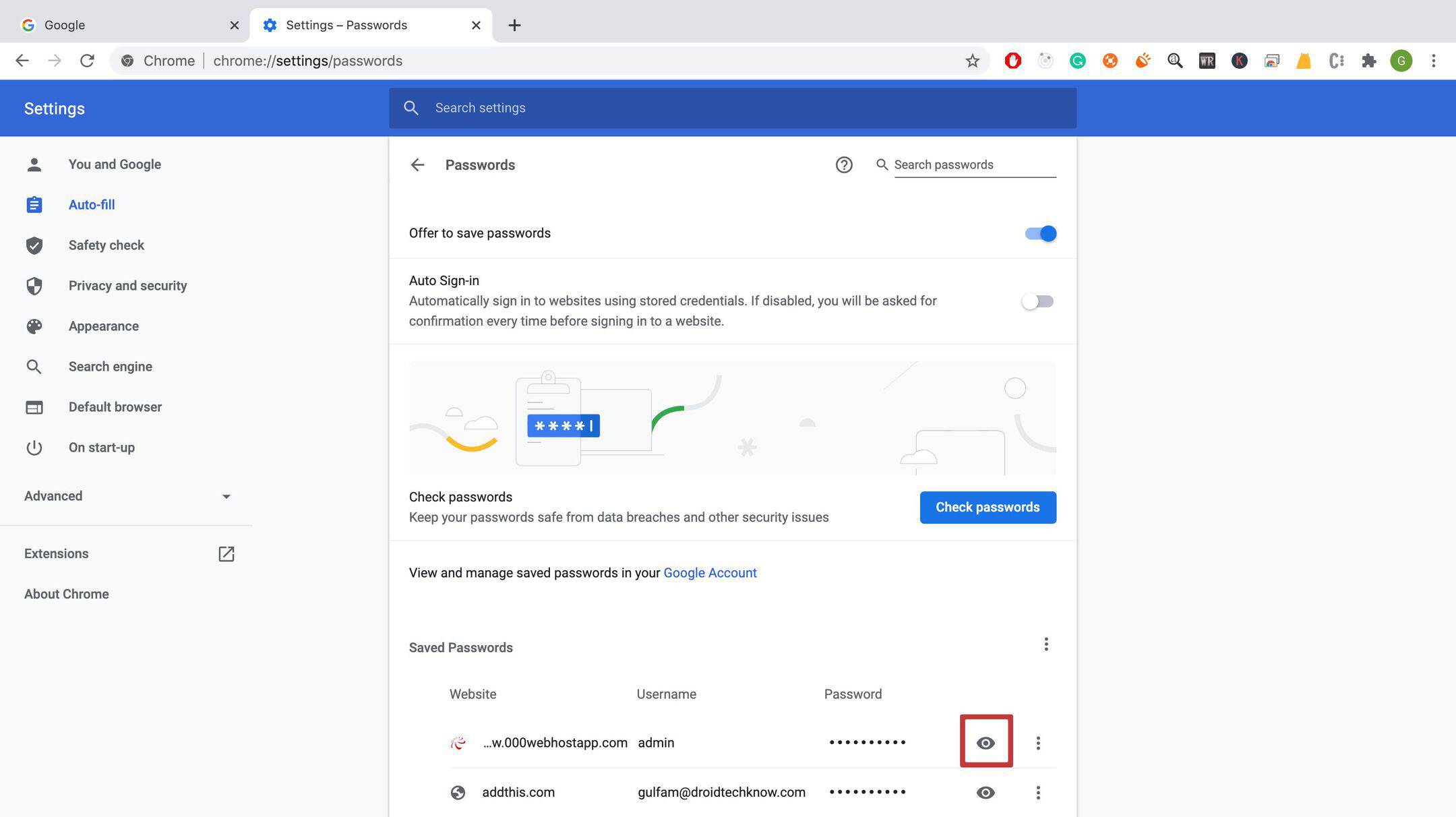The screenshot displays the Google Chrome settings page, specifically focused on the password management section.

At the top of the screen, a long gray bar spans across with the Google logo on the left, consisting of the word "Google" next to a multi-colored circle (red and green colors prominently visible). To the right of this logo, there's a search bar area accompanied by a blue gear icon labeled "Settings," followed by the word "Passwords."

Directly below this top bar, a blue search bar area is visible, displaying the text "Chrome" followed by a small vertical line and the URL "chrome://settings/passwords." To the right of this URL, there are various app icons in different colors and shapes (red, green, orange, yellow, and another green icon).

On the left-hand side of the screen, a sidebar menu in blue lists multiple configuration options. From top to bottom, they include "Settings," "You and Google," "Autofill" (highlighted in blue), "Safety Check," "Privacy and Security," "Appearance," "Search Engine," "Default Browser," and "On Startup."

In the main content area, the title "Passwords" is displayed at the top with a left arrow icon preceding it. Below the title, there's a search bar labeled "Search passwords" and an "Add" button. This section also features a blue bar with four asterisks (* * * *) indicating hidden or protected passwords. 

Finally, the bottom part of the screen shows a blue rectangle button labeled "Check passwords," prompting users to verify the security of their stored passwords.